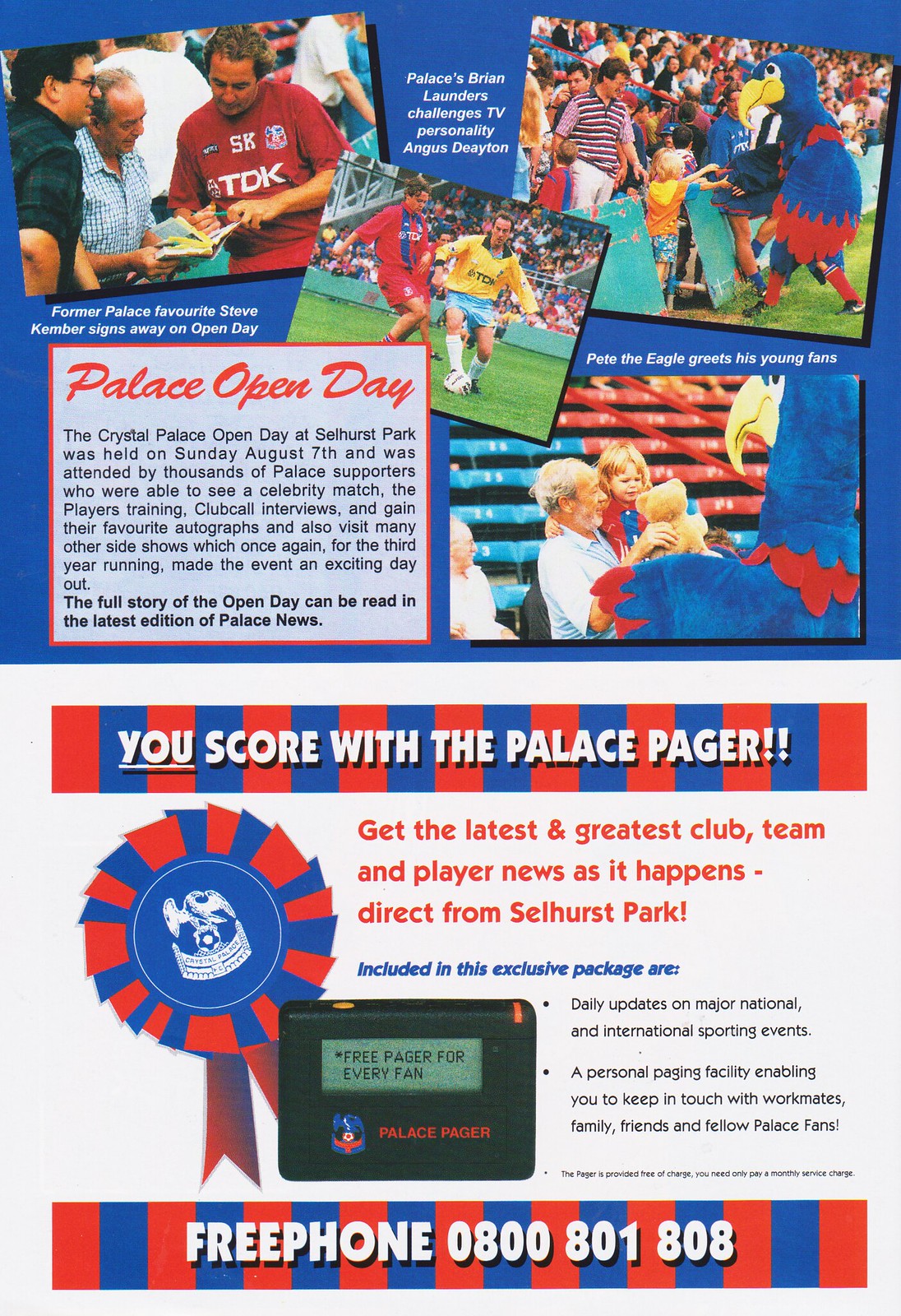This detailed page from a colorful game day program highlights Palace Open Day at Selhurst Park, held on Sunday, August 7th. The top half of the page features a recap of the event, showcasing a variety of photographs capturing different moments. Among these images, the central photo depicts two soccer players battling for the ball. To the left, a player is seen signing an autograph for a fan. On the right, the club’s blue bird mascot is captured greeting and shaking hands with a young supporter; a close-up of this interaction is displayed below.

The text accompanying these vibrant photos states: "The Crystal Palace Open Day at Selhurst Park was held on Sunday, August 7th, and was attended by thousands of Palace supporters who were able to see a celebrity match, the players training, club call interviews, and gain their favorite autographs, and also visit many other sideshows, which once again, for the third year running, made the event an exciting day out."

The bottom half of the page transitions into a colorful advertisement for the Palace Pager, which features a blue and red striped banner proclaiming, "You score with the Palace Pager." Below the banner, a ribbon encircles an image of the device, accompanied by text promoting its service: "Get the latest and greatest club, team, and player news as it happens. Direct from Selhurst Park. Included in this exclusive package are daily updates on major national and international sporting events, a personal paging facility enabling you to keep in touch with workmates, family, friends, and fellow Palace fans." The ad concludes with a banner instructing readers to "Free Phone 0800 801 808" to subscribe.